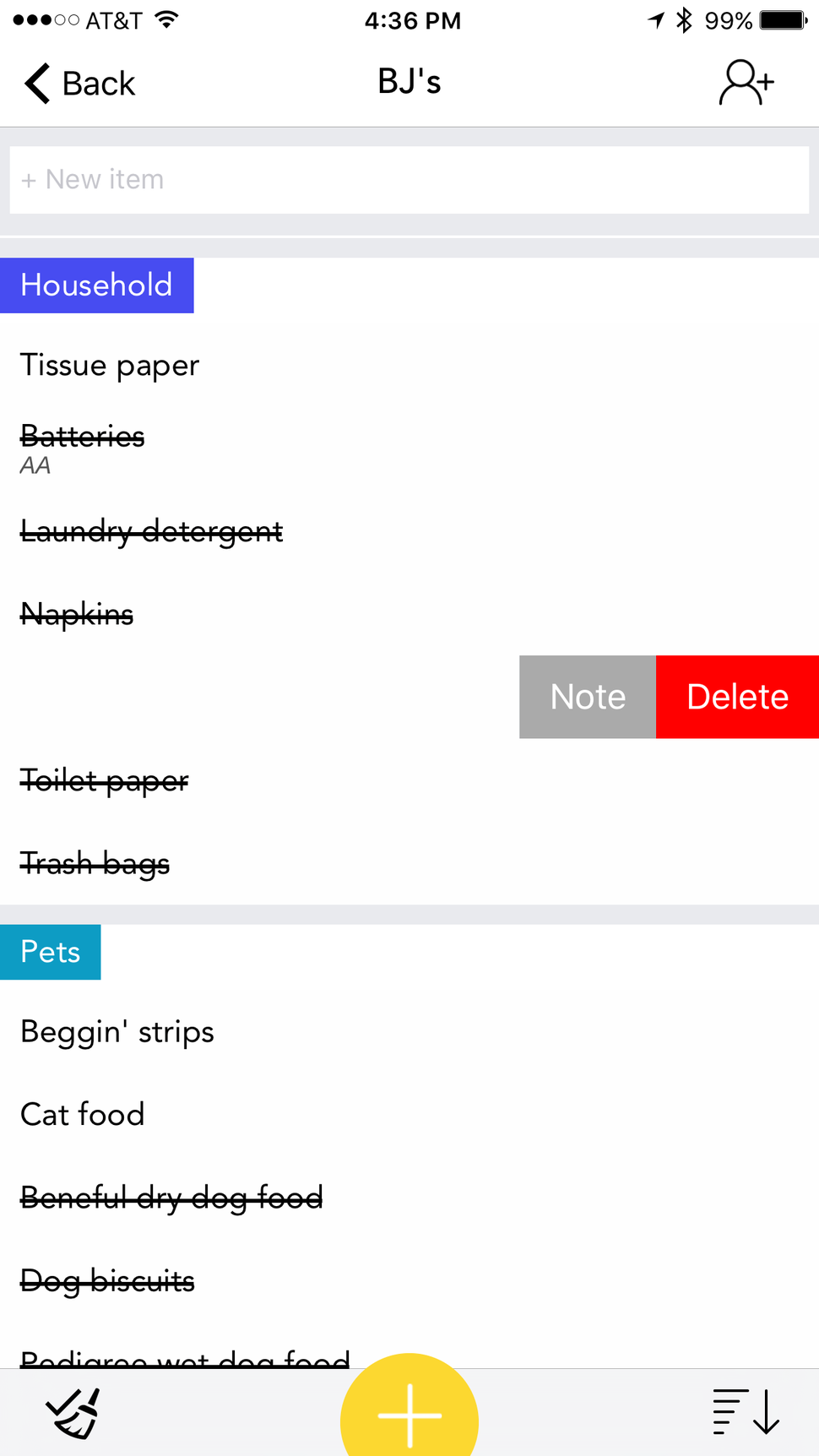**Detailed Caption of the Shopping List Screenshot:**

The screenshot displays a shopping list on a mobile phone with a white background and black text, recorded at 4:36 PM, as indicated in the status bar at the top. The status bar shows three out of five circles filled for signal strength under the AT&T carrier, a Wi-Fi strength indicator, a location arrow, a Bluetooth icon, and a battery status at 99% with a nearly full battery icon.

Below the status bar, the navigation bar features a back arrow with the text "Back" on the left, the title "BJ's" in the center, and a profile icon with a plus sign on the right. Beneath this is a gray bar with a white box labeled "Plus new item."

The shopping list is divided into two categories: "Household" and "Pets." The "Household" section, marked by a blue background with white text, includes:
- Tissue paper (without a strikethrough, implying it hasn't been checked off)
- Batteries (with a note indicating "AA")
- Laundry detergent
- Napkins (highlighted with a gray "Notes" button and a red "Delete" button beside it, without a strikethrough, suggesting it’s selected but not checked off)
- Toilet paper
- Trash bags

All items except for tissue paper and napkins have a strikethrough, indicating they’ve been checked off.

The "Pets" section, marked by a teal background with white text, lists:
- Beggin' Strips
- Cat food
- Benniple dry dog food
- Dog biscuits
- Pedigree wet dog food

All items except for Beggin' Strips and cat food have a strikethrough, indicating they’ve been checked off.

At the bottom of the screen is a gray bar with three icons:
- On the left, a black outline of a broom with a checkbox, which likely represents completion of tasks.
- In the center, a mostly circular yellow button with a white plus sign in the middle, possibly for adding new items.
- On the right, a filtering icon that might allow filtering in descending order, resembling common filter icons in word processing programs.

This detailed description captures the structure and function of each element displayed in the shopping list screenshot.